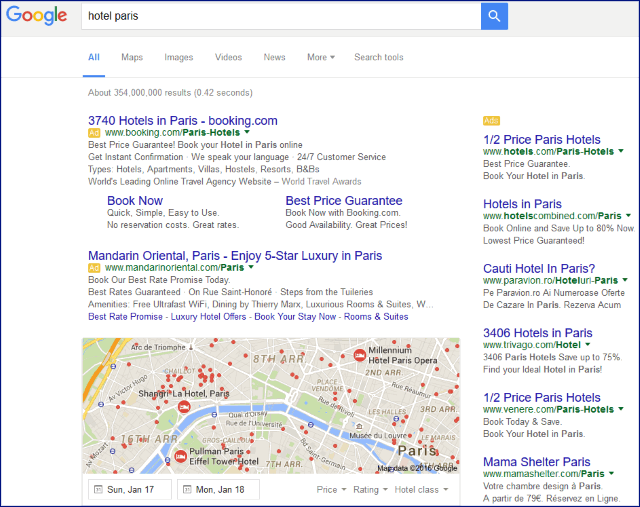A Google search result page is displayed with the query "hotel Paris." The results show 387,440 hotels listed, with the top result being the Mandarin Oriental Paris, indicating a luxurious five-star hotel option. Beside the primary results, a map highlights the locations of the returned hotels, marked with gold "ad" logos signifying sponsored content. On the right side, there is a sidebar filled with additional advertisements for various other hotels in Paris. The standard Google interface is present, featuring a white background, the Google logo at the top, and a search bar beneath it.